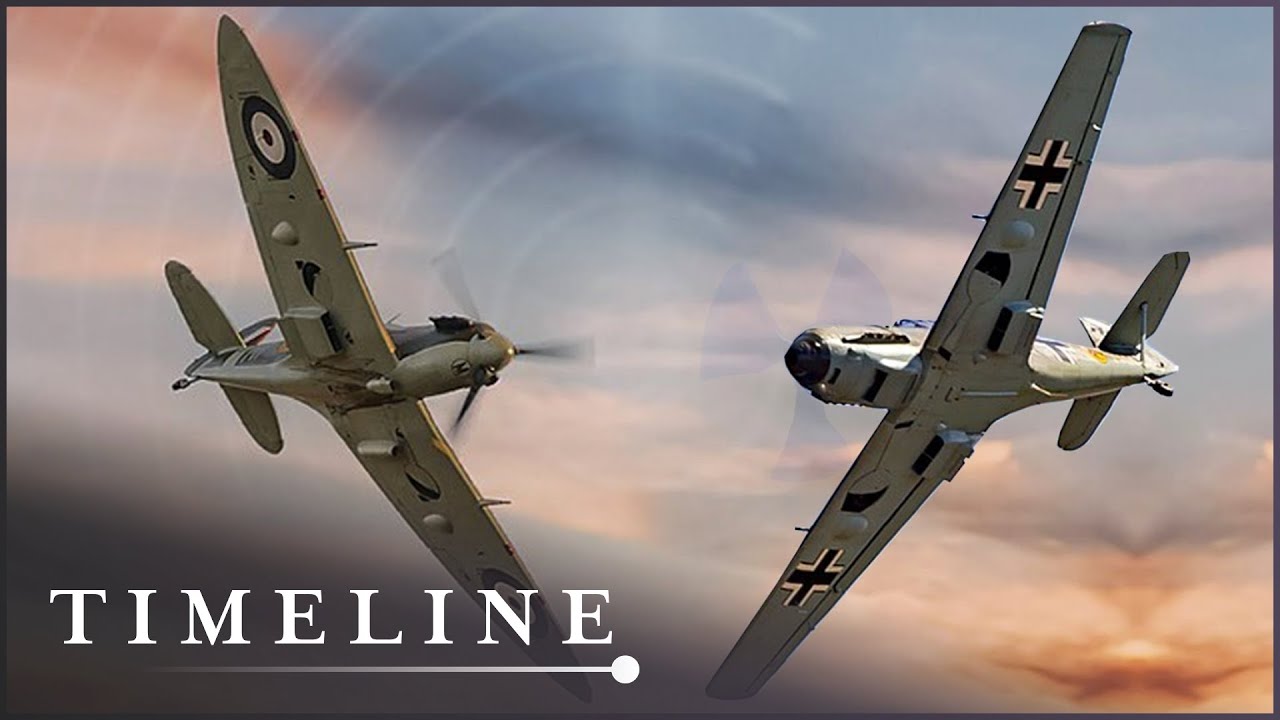This poster depicts two World War II fighter jets flying towards one another at a tipped angle, showcasing the undersides of their wings. The left jet features a roundel insignia with a dark circle, a light inner circle, and a dark dot at the center, while the right jet displays a black iron cross. Both steel gray planes are operated by propellers and soar high in the sky. The backdrop is a striking blend of gray and salmon hues with a hint of rust orange in the bottom right corner. Notably, the left fighter plane has an aggressive snarl painted on its nose. In the bottom left corner of the poster, against a dark gray background, the word "Timeline" is prominently displayed in white lettering with a white line underneath. The composition suggests a dramatic mid-air encounter, though it may be an artistic rather than a historical representation.